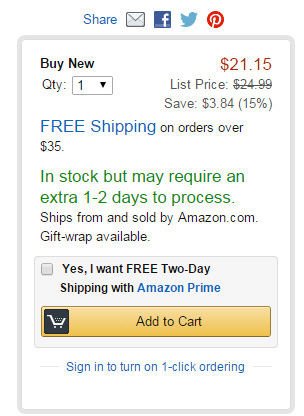This image is a detailed snapshot of a purchase and shipping description from Amazon.com. It highlights that the item, originally priced at $24.99, is on sale for $21.15. Additionally, the image indicates that buyers can enjoy free shipping on orders over $35. It confirms the item is currently in stock, but notes that it may require an additional one to two days for processing. The item is both shipped and sold by Amazon.com. At the bottom of the image, there is an option to add the item to the cart. Above this, another option with an unchecked checkbox states, "Yes, I want free two-day shipping with Amazon Prime." At the very bottom, a blue link encourages users to "Sign in to turn on 1-Click ordering."